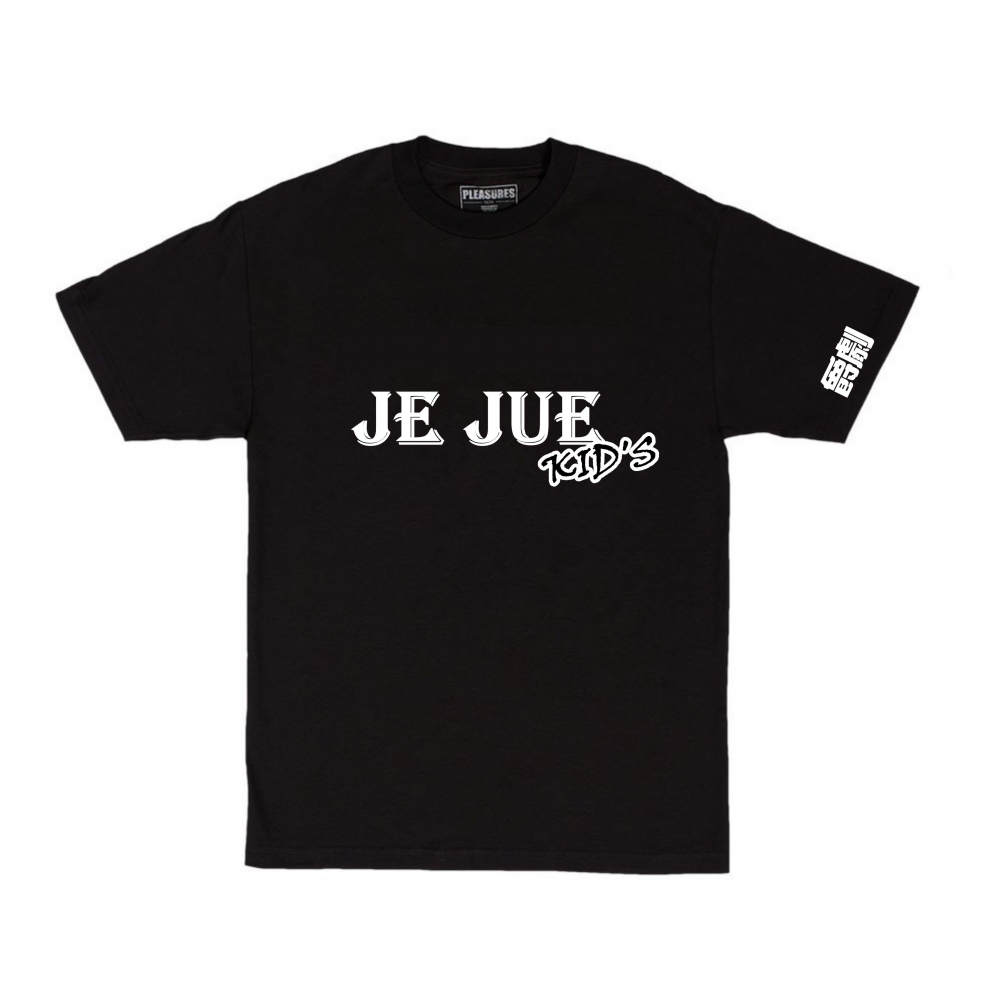The image depicts a black t-shirt set against a plain white background, positioned as though it were worn, with sleeves extended and lying flat but upright. The shirt features a small white tag along the inside neckline, which reads "pleasures" in white letters on a black background, outlined in white. Centrally positioned on the chest area, the shirt showcases large, bold white letters spelling "J-E-J-U-E" horizontally, with the word "kids" written diagonally in black letters with a white outline, located just beneath the final "E." Additionally, the left (or right, depending on orientation) sleeve contains an unreadable white design or Chinese characters, outlined in black, adding an extra element of detail to the shirt. The photo's minimalist setting emphasizes the t-shirt, making it the sole focus of the image. This appears to be a children's t-shirt, likely for a brand named "Juju's Kids."